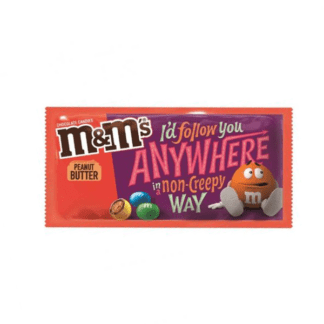This image depicts a package of Peanut Butter M&M's candy against a solid white background. The packaging predominantly features a striking blend of red and orange hues, while a prominent purple banner stands out in the middle to the right side. The purple banner showcases the playful, colorful message: "I'd follow you anywhere in a non-creepy way". The text is creatively designed with "I'd" and "you" in white, "follow" in orange, "anywhere" in large, bold, pink letters, with "in" and "way" in white and "non-creepy" in orange.

The top left corner of the package features the iconic M&M's logo and a label indicating the peanut butter flavor in an outlined orange section with brown letters. Beneath the banner, the orange M&M mascot, known for his scared expressions, is prominently displayed. This character is seen on the lower right-hand side, with wide, apprehensive eyes looking to the right, a half-open mouth, a white "M" on his tummy, and sporting white gloves and shoes. The background behind this mascot and the package contains a mix of bright colors such as turquoise, green, yellow, and brown, reminiscent of the colorful imagery you'd expect from a candy associated with a whimsical theme like the Willy Wonka movie.